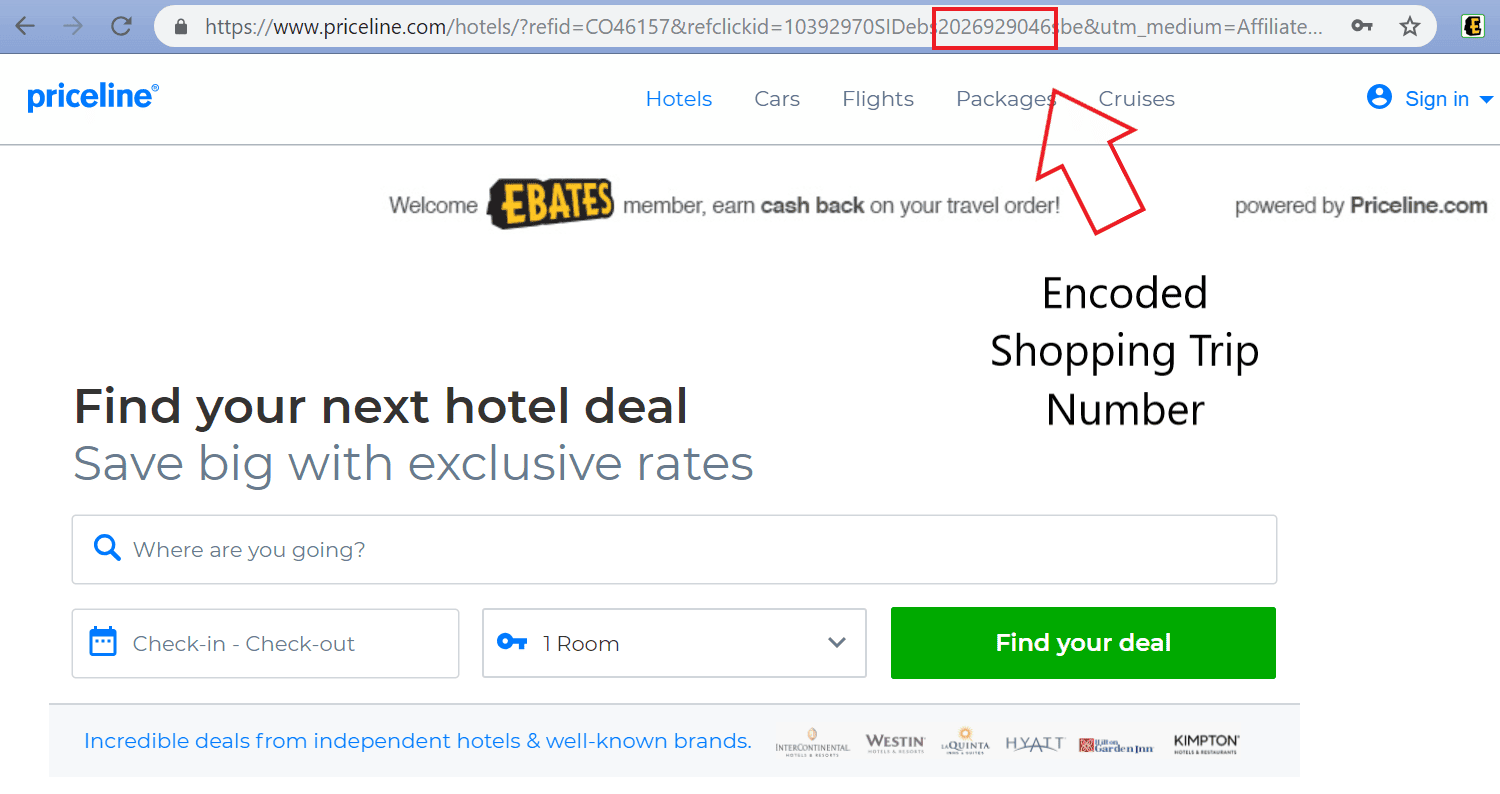A screenshot of the Priceline.com website, showcasing a segment focused on hotel bookings. The interface has a clean white background. At the top, there's the URL displayed prominently: "Priceline.com/hotels/?REFID=", followed by a string of letters and numbers, "2026929046", emphasized with a red rectangle around it. The words "Priceline Hotels" appear in blue, while other menu options like "Cars", "Flights", "Packages", and "Cruises" are in gray. 

An eye-catching red arrow points to the red rectangle with the number. The top right corner of the screen features a user-specific message: "Sign in, Welcome eBates member", highlighting the benefit of earning bolded "cash back" on travel orders. The eBates logo appears in bubble letters, denoting it as a partner powered by Priceline.com.

Below the arrow, there's an "Encoded Shopping Trip Number" indicating a specific booking session. Beneath this, a call-to-action invites users to "Find your next hotel deal". Promoting savings, the page suggests users can "Save big with exclusive rates". 

A search bar facilitates the booking process, flanked by a calendar input for check-in and check-out dates. Other details include a key symbol showing the selection of "1 Room". A prominent green rectangle labeled "Find Your Deal" encourages users to commence their search.